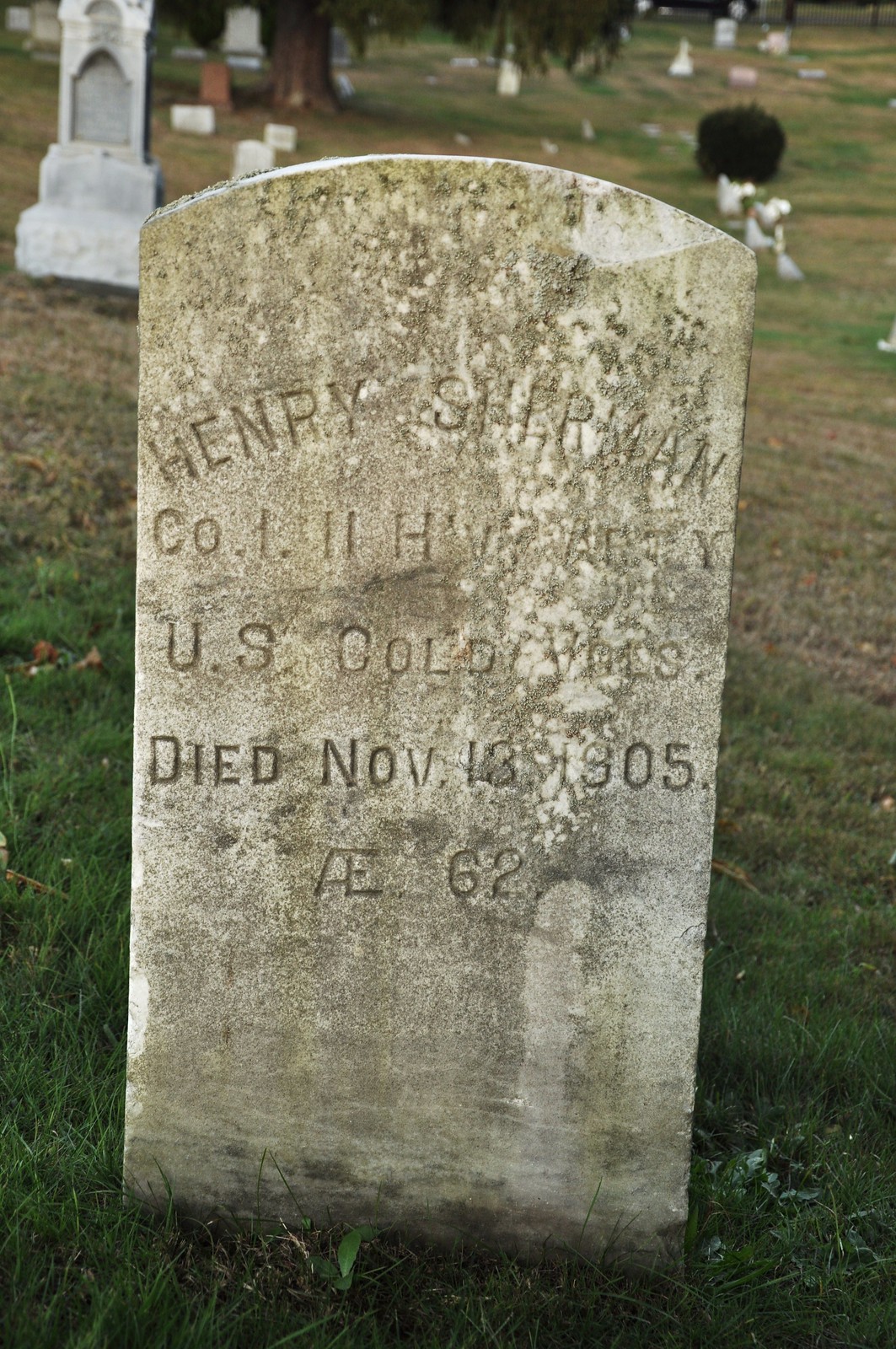The image depicts an aged, weathered headstone made of concrete, covered in greenish algae and darkened with age, situated in a cemetery during the daytime. The headstone features the name "Henry Sherman" prominently inscribed at the top, followed by an inscription indicating his association with the army, which is partially legible as "Co-1-2 U.S. Cold something." Below this, the headstone records his death on November 13, 1905, and his age at death as 62. The overgrown grass at the base of the headstone, along with various other mossy stains, highlights its antiquity. In the background, the cemetery extends into a grassy field dotted with headstones of varying sizes and types, a shrub, and a large pine tree. The scene conveys a serene yet solemn atmosphere.